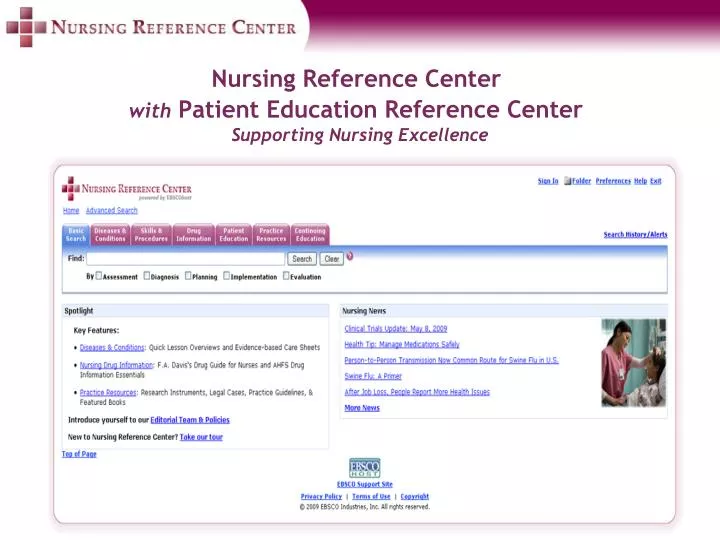This image depicts a comprehensive web page from a Nursing Reference Center. In the top left corner, there's a recognizable medical symbol, often referred to as a cross, indicating a healthcare-related site. To the right of this symbol, the title "Nursing Reference Center" is prominently displayed. Adjacent to this title is a purple banner with a gradient design, transitioning to white as it moves downward.

Underneath the banner, the site underscores its purpose with the phrases "Nursing Reference Center" and "Patient Education Reference Center," emphasizing its role in supporting nursing excellence. Below this, the main body of the web page reveals a user-friendly interface designed to provide a wealth of information.

The top section of the navigation menu includes several tabs allowing users to access detailed information on topics such as Diseases and Conditions, Skills and Procedures, Drug Information, Patient Education, Practice Resources, and Continuing Education. Additional resources are available below these tabs, suggesting further clickable options for users seeking extensive nursing-related knowledge. The overall design conveys a structured and in-depth resource center aimed at enhancing the professional knowledge and skills of nurses.